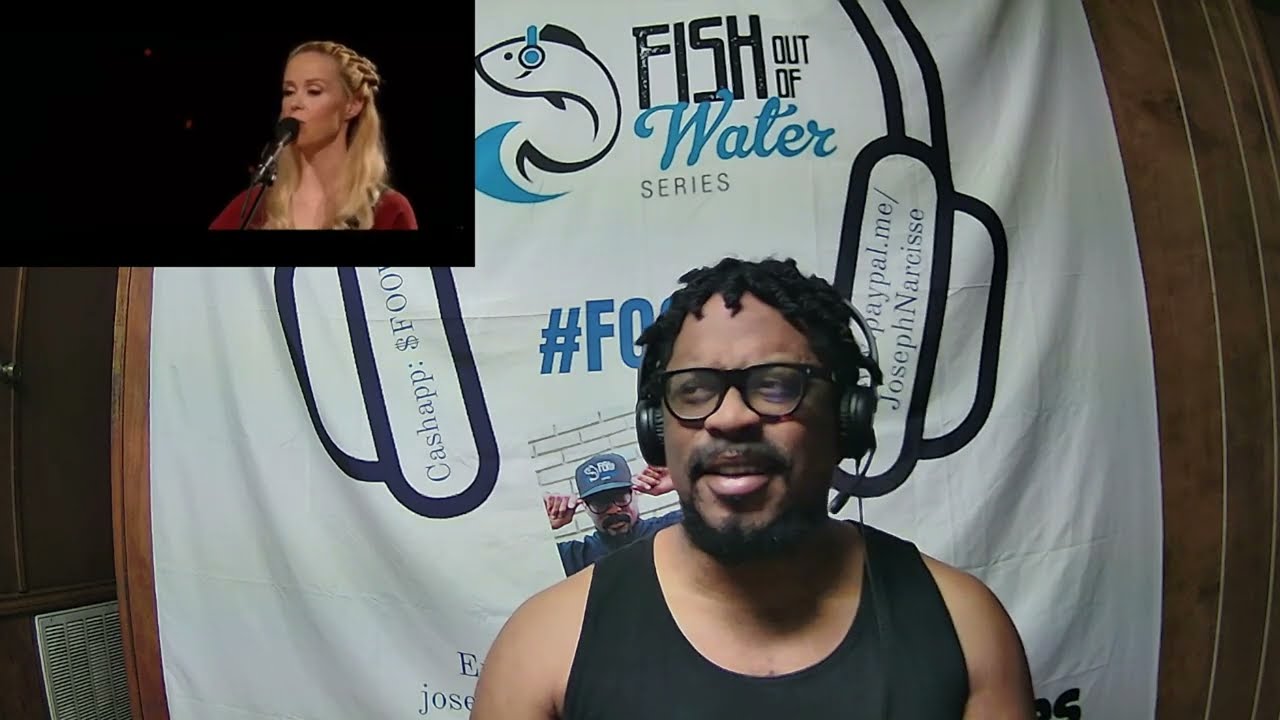In the image, a man with short curly black hair, black-framed glasses, a mustache, and a beard on his jawline is prominently positioned at the bottom center. He wears a black sleeveless t-shirt and appears to be staring towards the left. The man is equipped with a headset. Behind him, there's a board framed in brown, featuring a white fabric background. On this fabric, a fish logo and the text "Fish Out of Water Series" are visible. Additionally, there are logos for PayPal and Cash App links, specifically "PayPal.me/JosephNarcisse." In the top left corner of the image, a split screen displays a woman in a red shirt singing into a microphone. The scene appears to be set indoors, with various colors such as black, tan, red, brown, gray, white, purple, light blue, and blue enriching the image. Overall, it gives the impression of a man reacting to a live music performance.